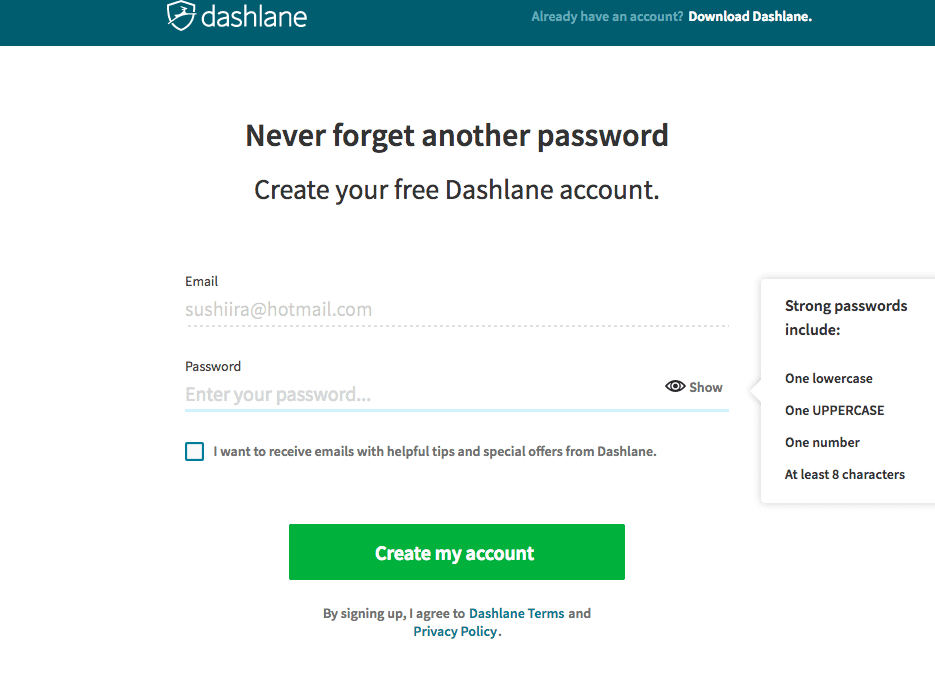This image from the Dashlane website features a sleek, dark greenish-blue rectangular interface designed for user account creation and downloading the Dashlane software. 

At the top of the rectangle, there is an icon of a deer leaping through a shield, representing the Dashlane logo. Below this, the text reads, "Already have an account? Download Dashlane," prompting existing users to access the download link.

Further down, a bold statement encourages users, "Never forget another password," followed by a call-to-action, "Create your free Dashlane account." This section begins the account creation form. 

The first input field is labeled "Email," showcasing an example email address (sushiira@hotmail.com) in grayed-out text to guide users. Following this is another input field for "Password," featuring placeholder text ("Enter your password..."). Adjacent to the password field is an eyeball icon labeled "Show," which users can click to reveal the typed password. A note beneath this emphasizes that strong passwords should include one lowercase letter, one uppercase letter, one number, and be at least eight characters long.

Beneath the password field is a checkbox option for users to opt in to receive emails with helpful tips and special offers from Dashlane.

At the bottom of the interface, a prominent green rectangular button with white text invites users to "Create my account." Below this button, in smaller black text, is a disclaimer stating, "By signing up I agree to Dashlane Terms and Privacy Policy," with "Dashlane Terms" and "Privacy Policy" appearing as blue hyperlinks, likely leading to the respective documents.

The image effectively communicates both the value proposition of Dashlane and a clear, user-friendly process for new account creation.